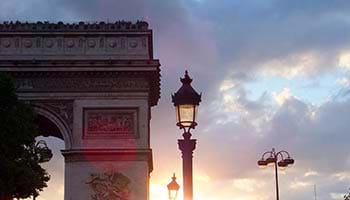This photograph, taken in a landscape orientation, captures a dusk or dawn scene in Paris, featuring the famous Arc de Triomphe prominently in the background on the left side. The arch, notable for its large columns and ornate carvings, appears partially obscured but still recognizable. The centerpiece of the image is a vintage-style street lamp, made of cast iron with spires and decorative elements, which is lit, casting a warm glow that complements the natural lighting of the scene. Flanking this central lamppost are two additional street lamps—a modern one on the right and another antique one in the bottom left corner. The street lamps take precedence in the composition, creating an interesting contrast with the monumental arch behind them. The sky overhead is a tapestry of cloud coverage intermingled with patches of blue, tinged with colors of sunset or sunrise—shades of orange, pink, and gold. To the left, the outline of a tree is visible, partially shrouded in shadows. The image does not include people or text, focusing solely on the interplay of these architectural and natural elements.